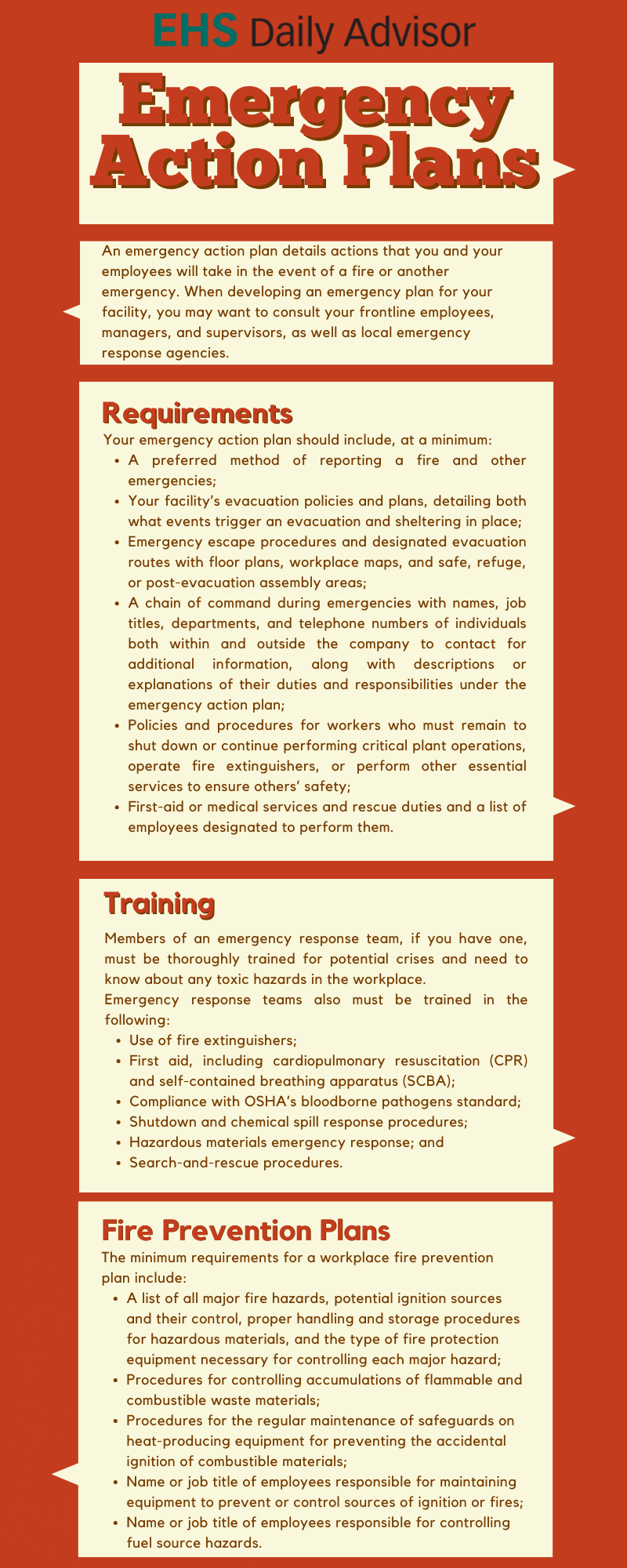The image is a detailed poster from the EHS Daily Advisor titled "Emergency Action Plans." The poster features a copper-orange background with matching upper letters and is bordered in red. The primary title, "Emergency Action Plans," is displayed prominently at the top in bold red letters. Below the title, the poster is segmented into several ivory or beige rectangles that are filled with information in small, red text, making some of the fine print difficult to read.

The first section introduces the emergency action plan, emphasizing the importance of detailing actions for employees to take in incidents such as fires or other emergencies. This section likely suggests consulting frontline employees, managers, supervisors, and local emergency response agencies when developing the plan.

The subsequent sections are divided into specific categories: "Requirements," "Training," and "Fire Prevention Plans," each detailed in their own rectangles with bullet points outlining key aspects of each category. "Requirements" appears to have five bullet points, "Training" contains five or six, and "Fire Prevention Plans" also includes five bullet points. The poster is long and slender, providing comprehensive but densely packed information on emergency procedures aimed at ensuring workplace safety.